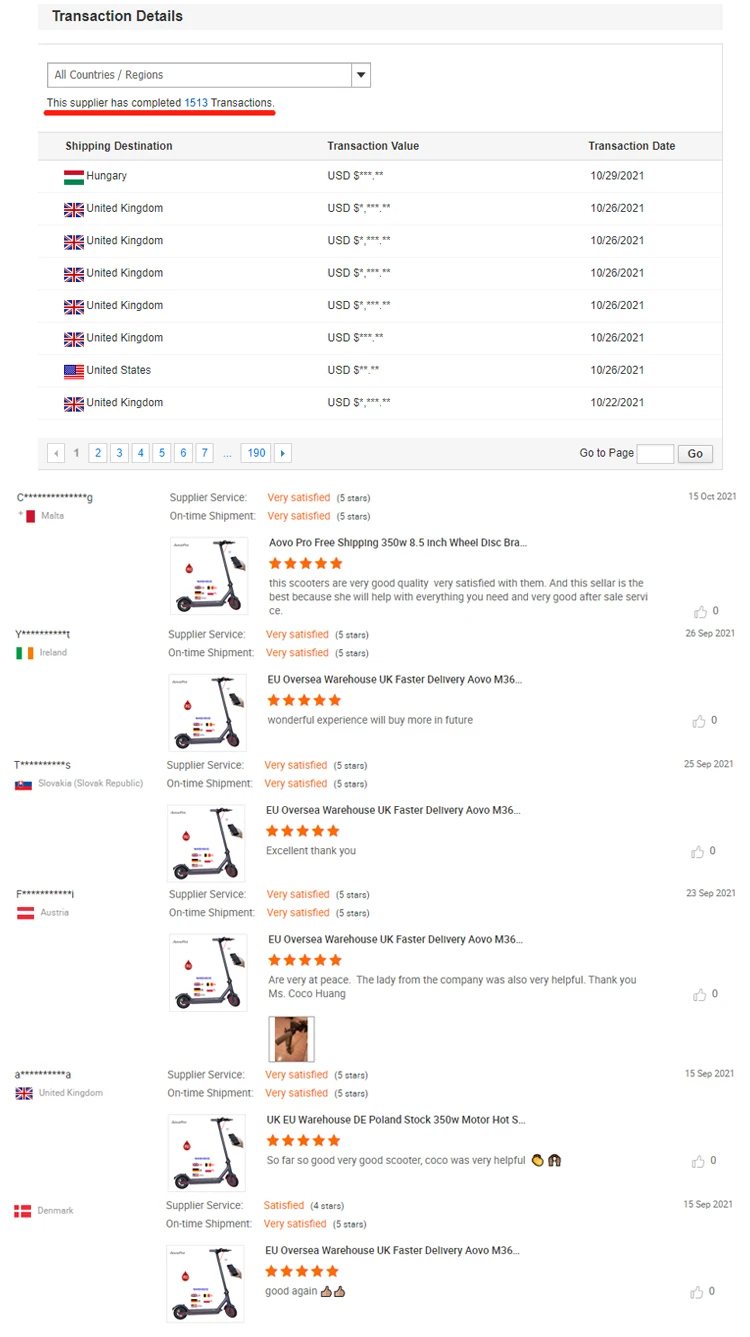This screenshot captures a webpage displaying transaction details on a white background. In the upper left-hand corner, the title "Transaction Details" is prominently featured. Just below the title, at the page's upper section, there is a drop-down menu labeled "All Countries/Regions," underlined in red. Adjacent to this, the text "This supplier has completed 1,513 transactions" is visible. 

Following this introductory section, there is a detailed listing of individual transactions. Each transaction entry includes the shipping destination represented by a national flag, the transaction value, and the transaction date. Towards the bottom of this section, there is a navigation interface comprising a series of page buttons that allow the user to scroll through the transactions. Additionally, there is a "Go to page" input box accompanied by a "Go" button to jump directly to a specific page.

The transaction details are organized in rows, with each row containing several columns of information. The left-hand column provides the flag of the shipping destination and what is likely the seller's name. Adjacent to this column, there is a photograph depicting a black scooter, indicative of the items bought or sold. Each item is labeled, and there is a consistent display of five orange stars, suggesting high customer ratings. On the far right side of the page, there is additional information indicating the number of thumbs up the transaction received and the date of the transaction.

Such a layout provides a detailed and organized view of multiple transaction records, ensuring the user can easily navigate and assess past transactions.